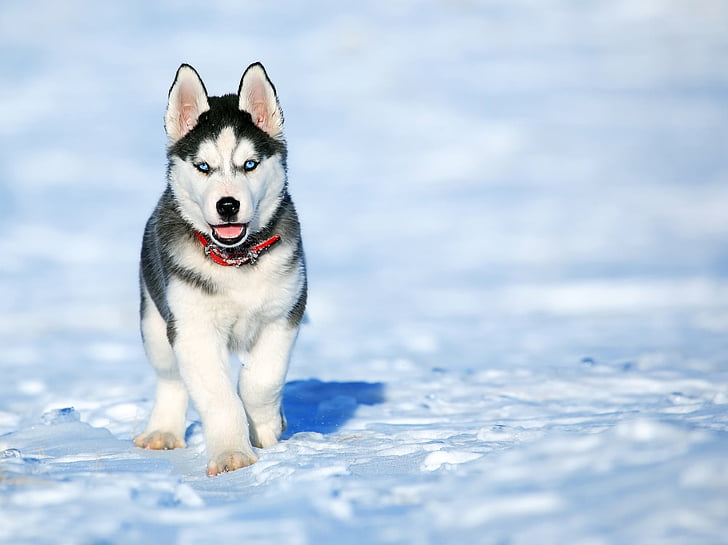The image features a young Siberian Husky puppy prominently positioned on the left side, walking directly towards the camera across an expansive, flat, snow-covered plain. The Husky displays striking white fur with a mix of black and grey over its back, and distinguished black markings on the top of its head, ears, and back. Its sharp, bright blue eyes shine brilliantly, adding to its alert and engaging appearance. Both of its pointed ears stand straight up like radars, and its shiny black nose is clearly visible above its slightly open mouth. The puppy is adorned with a vivid red collar, enhancing its standout look against the snowy backdrop. The entire landscape, stretching endlessly around the puppy, is a vast field of icy blue and white, indicating a bright and sunny day. The snow plain is featureless, enhancing the pup’s presence as it casts a defined shadow towards the right and behind it.